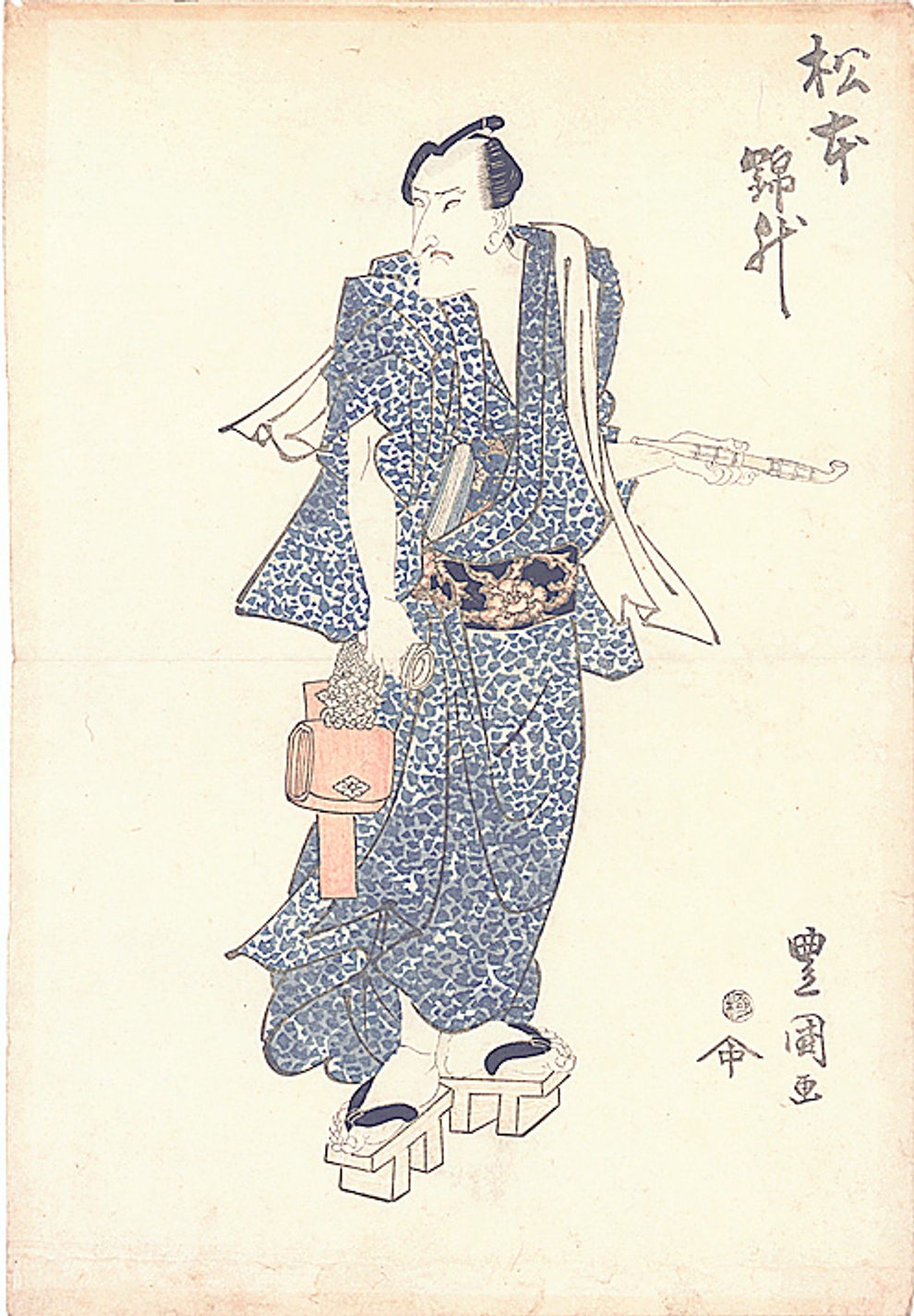This image is a detailed drawing or painting of an Asian person, likely intended to be the central focus. The person is dressed in a flowing blue gown adorned with white and gold accents and a blue and white paisley patterned belt. They have a white scarf draped over one shoulder. The individual is holding a brown-tinted purse in the right hand and a possible instrument in the left hand, though the exact object is indistinct. They have slicked-back hair and a mustache, suggesting a male appearance, but the presence of the purse lends some ambiguity to their gender. They are standing in blue platform sandals, shaped like two T-forms at the bottom. The person is gazing to the left. The background is plain, with no additional elements, and there is Asian, likely Chinese, text on both the top right and bottom right corners of the image. The entire artwork is set against a white sheet with a tan border. The colors prominently featured include blue, white, gold, brown, pink, tan, and off-white.